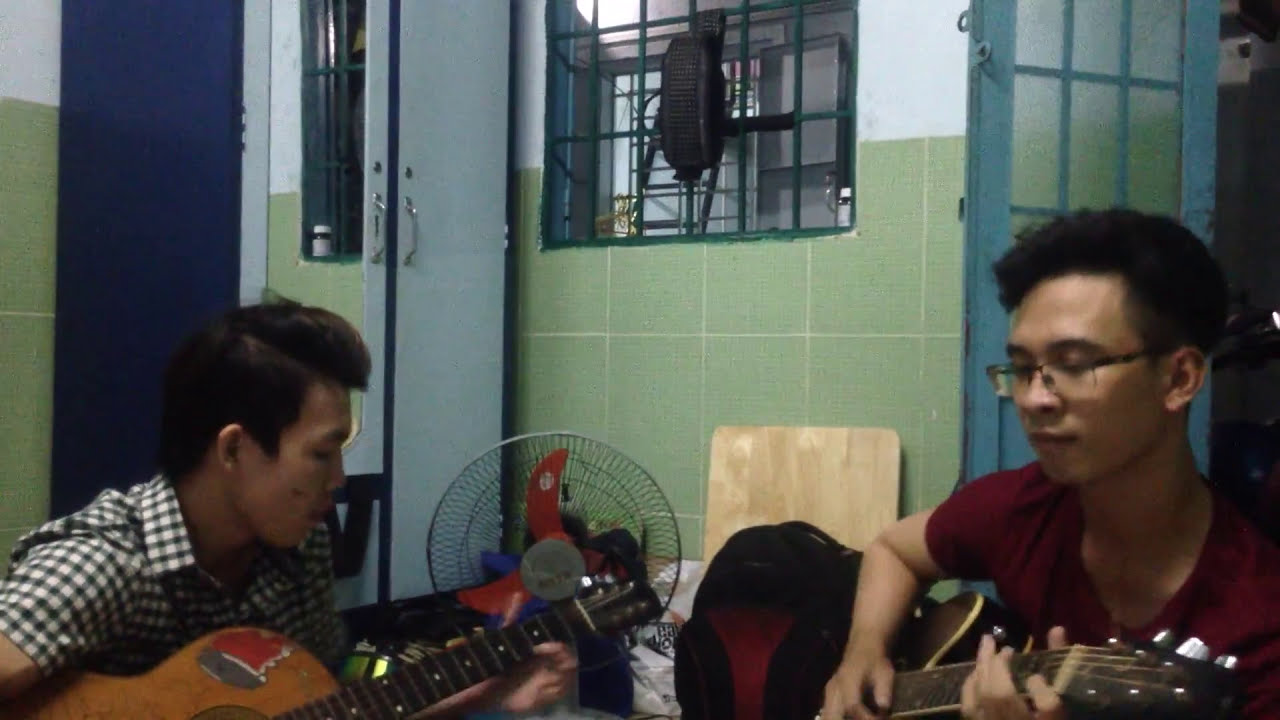The image depicts two young, Asian men in their early twenties playing acoustic guitars in a small room. The man on the left, situated in the lower part of the picture, wears a short-sleeved, black and white checkered collared shirt and is playing an older acoustic guitar with a sticker on its top right corner. The man on the right is wearing glasses and a dark red t-shirt while playing a newer, darker brown guitar. Both have dark hair. The room features a distinctive green-tiled wall with white grout, and the upper part of the wall is painted white. In the upper right corner, there's a blue door with a window panel. A floor fan with red and blue blades is situated between the two men. In the background, towards the middle-left side, there's a vertical white cabinet with a silver handle and a lock, extending from the floor up past the top of the image. Next to the cabinet is a strip of blue. The room's window has bars and is painted a bluish-green hue.